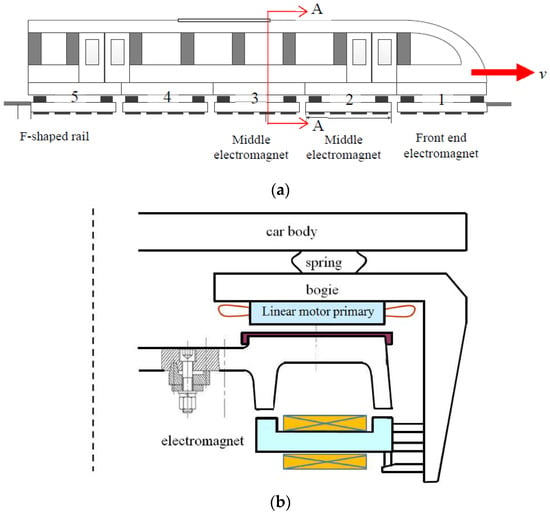The image is a vertical engineering drawing of an electromagnetic train, detailed in both an exterior view and a cross-sectional view. At the top, there's a forward-facing side view of the train car, headed to the right, marked with a red arrow indicating its direction. The train car is divided into five sections, numbered from front to back, with a letter A highlighting the cross-sectional area. Section 3, identified as the "middle electromagnet," intersects section A. The lower part of the image features the cross-sectional diagram, offering an intricate glance at the train's internal assembly. From the top down, the components are labeled: the car body, a pair of curved lines indicating the spring system, the bogie, the linear motor primary, and finally, the F-shaped magnetic rail beneath. This detailed diagram showcases the assembly and functional elements of the electromagnetic train, highlighting how it operates and maintains its glide along the magnetic rails.